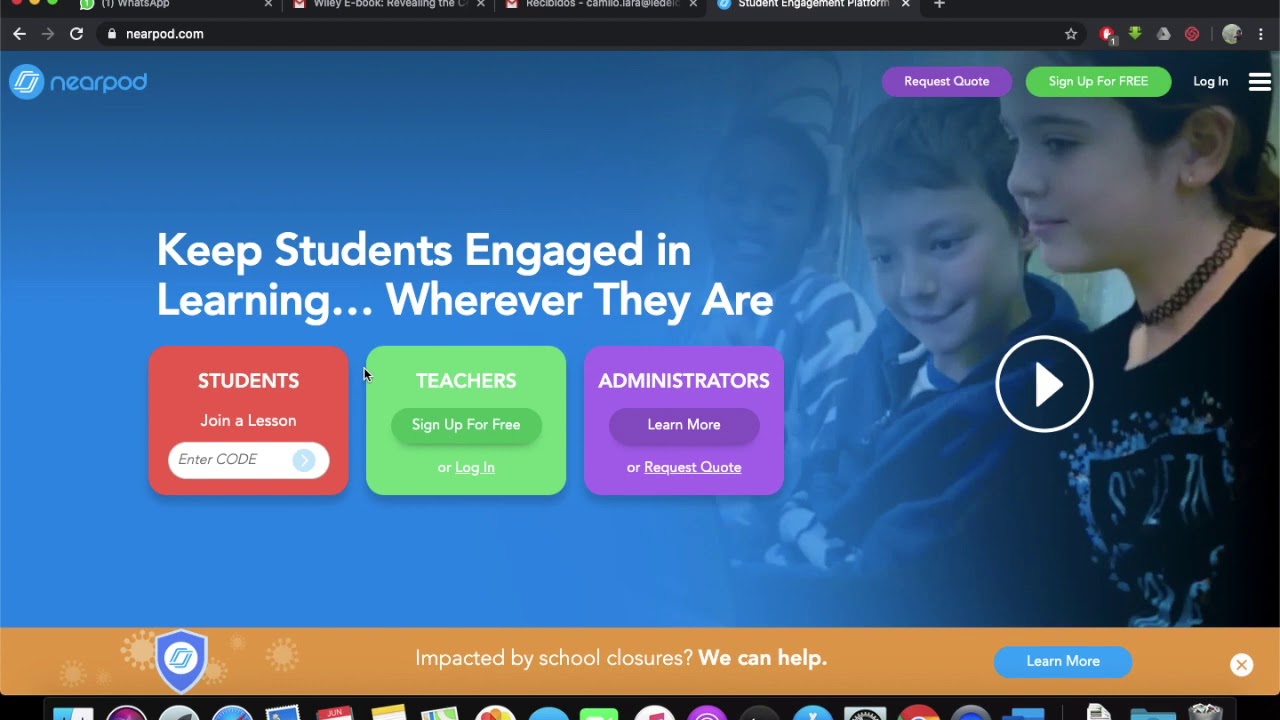Screenshot of the Nearpod website's homepage showcasing various navigation and interactive features. The top section prominently displays options such as "Request Quote," "Sign Up For Free," and "Log In," alongside a hamburger menu icon. The main banner reads, "Keep students engaged in learning wherever they are," emphasizing Nearpod's commitment to accessible education.

The interface also includes prompts for students to join a lesson by entering a code, while educators and administrators have highlighted options to "Sign Up For Free," "Log In," "Learn More," or "Request Quote." The terms "Request Quote" and "Log In" are underlined, indicating they are clickable hyperlinks.

At the bottom of the page, there is a notice addressing the impact of school closures, with a supportive message: "Impacted by school closures? We can help." This section contains a blue rectangular button labeled "Learn More" in white text, and a white circular icon with an 'X' for closing the message.

The background features a split design—blue on the left side and an image on the right side depicting three students, possibly engaged in a learning activity, suggesting an educational setting.